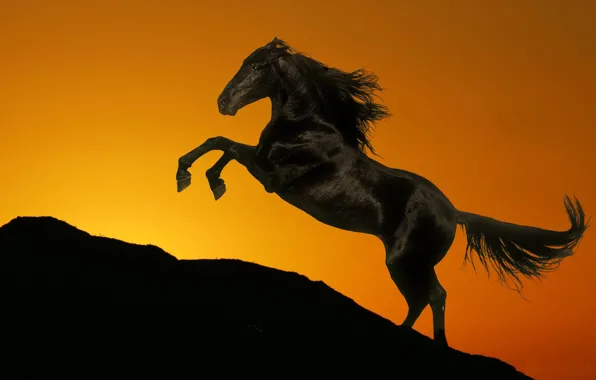The image appears to be a digitally altered photograph, rectangular in shape and horizontally oriented. At the bottom, a pitch-black hillside slopes gently upward. Above this hill, an orange glow, transitioning to yellow on the left side, suggests a sun setting behind the hill, although the sky looks more like an artificial backdrop than a natural sky. Dominating the scene is a black horse with shiny fur, positioned on the hill and facing left. The horse, which has characteristics of a Mustang or thoroughbred, is captured mid-rear on its hind legs, with its mane and long tail flowing backward, as if blown by the wind. Its ears are pinned back, adding to its dynamic and powerful stance. The hill is barren, lacking any foliage and emphasizing the stark contrast between the dark foreground and the luminous background.